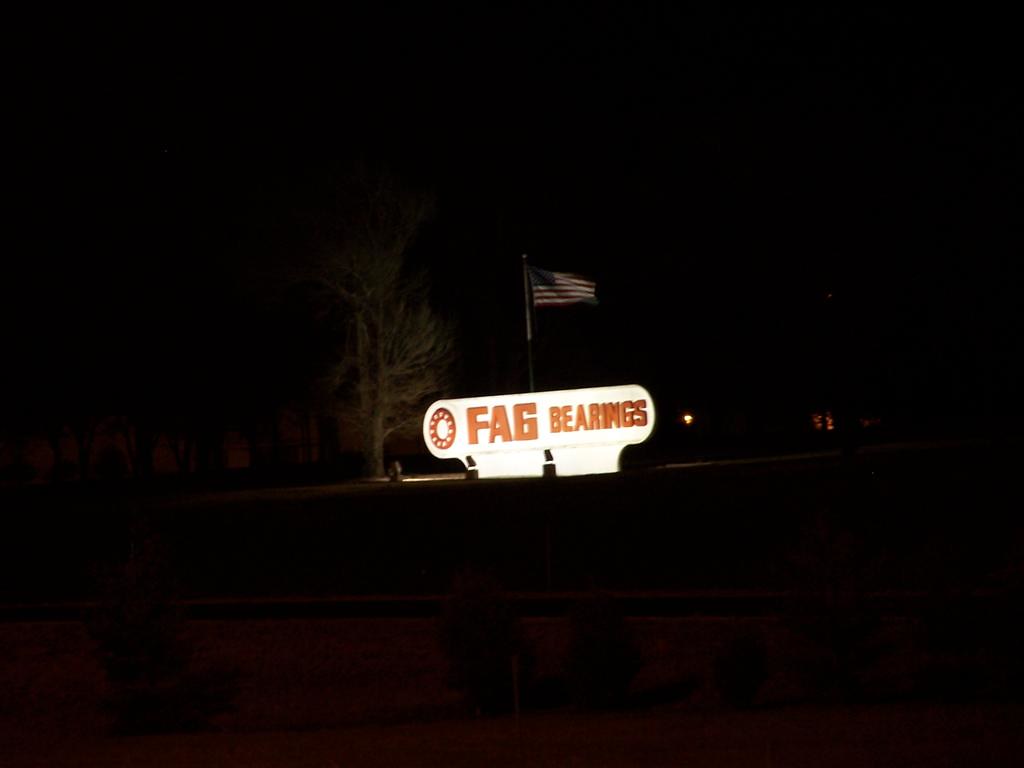This nighttime photograph, taken outdoors, is characterized by its deep darkness, rendering the sky a vast black void. The image predominantly features the silhouettes of trees against the night sky, with the dense, textured leaves suggesting evergreen or pine types. Central to the composition is a brightly illuminated LCD sign. This curved rectangular sign, casting light on its immediate surroundings, displays the text "FA6 Bearings" in bold orange letters, accompanied by an orange circle. The illumination from the sign also highlights a metal flagpole next to it, which proudly bears an American flag pointing to the right side of the image. Behind the sign, a tree stands out more clearly than the others due to the light, its green leaves visible. In front of the sign, roadwork cones and patches of grass and shrubbery can be noted, contrasting with the otherwise pervasive darkness. The overall scene suggests a location far from additional artificial light sources, with the sign's brightness being the primary light in the image.